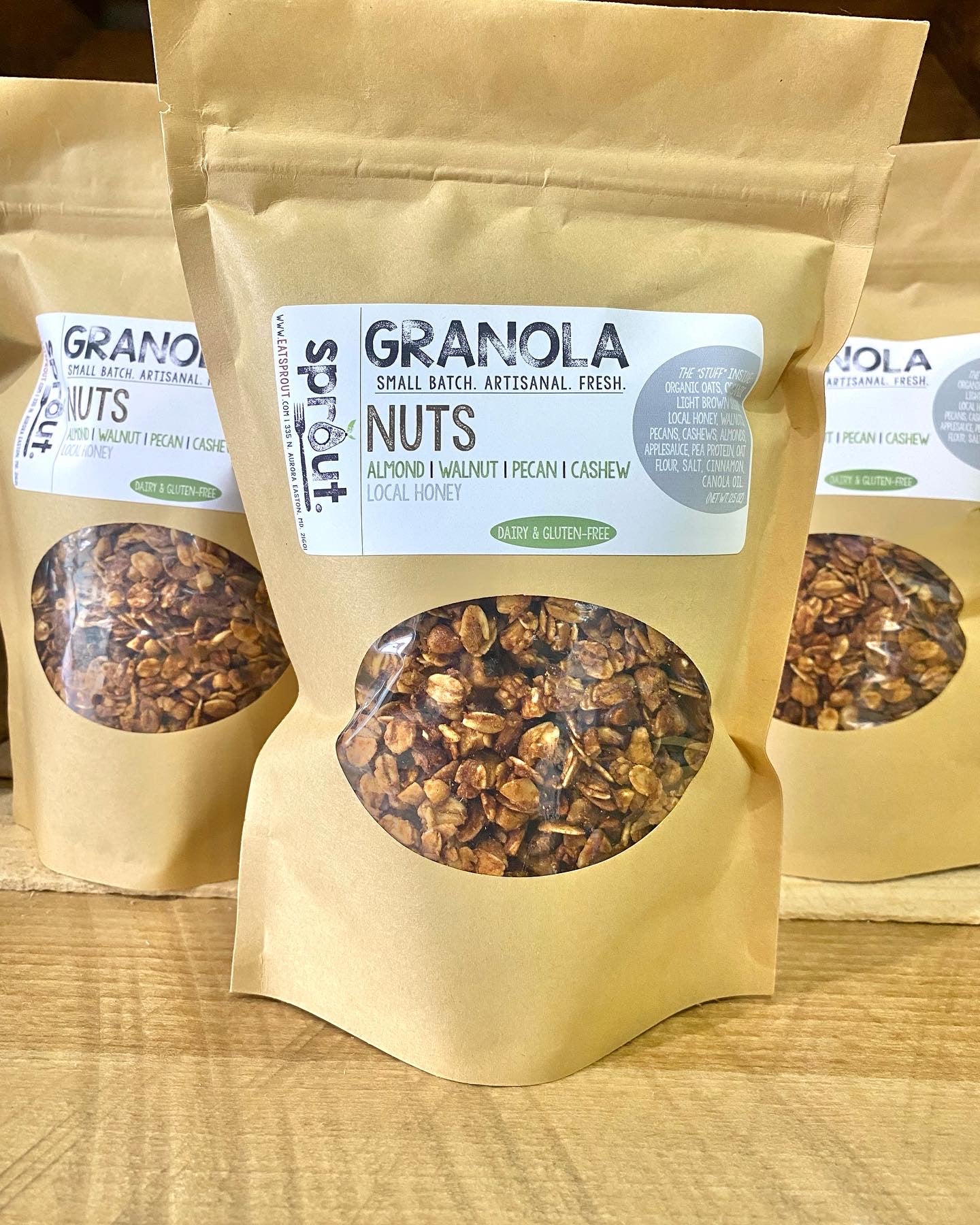The image showcases a close-up of three artisanal granola pouches arranged on a wooden tabletop, with one pouch in the front and two slightly off-center behind it. These pouches are made from a light brown, natural paper material, each featuring a resealable zip-top. Prominently displayed along the top of each pouch in large brown letters is the word "Granola," with the word "Nuts" written beneath it in a lighter brown font. Vertically aligned on the left side of the white label is the brand name "Sprout," next to the website www.eatsprout.com. The clear plastic window on each pouch reveals a mix of granola, including fresh nuts like almonds, walnuts, pecans, and cashews. The pouches also read "small batch, artisanal, local honey, dairy and gluten-free." While there is a silver label on the right side of each pouch, the text is too small and distorted to read clearly. The granola visibly contains oats and various nuts, reinforcing the product's artisanal and fresh appeal. The entire scene, though realistic, gives a slightly edited, almost photoshopped appearance against the wooden surface.